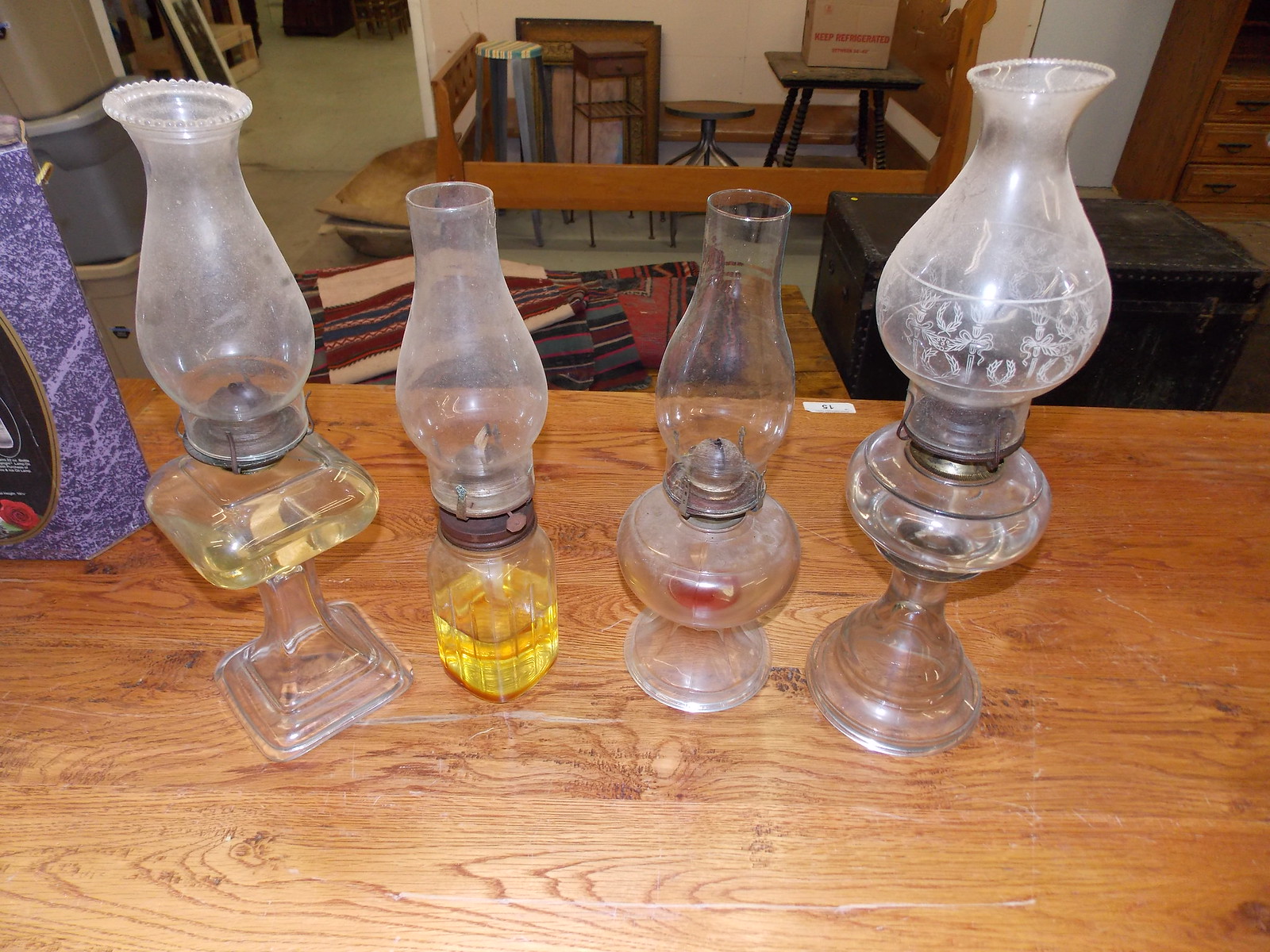This image features a set of four old, dusty oil lanterns arranged in a line on a light brown wooden table. The two larger lanterns at the outer ends frame two smaller, narrow ones in the middle. Each lantern holds a bit of oil at the base, with a noticeable light yellow tint. The lanterns, resembling kerosene glass bottles, have distinctive oval tops that curve to a slightly rusted metal section, which features a small circle, likely for the wick.

In the background, the scene is enriched by various types of antique furniture and decor. Notably, there are several nightstands and smaller tables, as well as a striped rug with colors of red, orange, light brown, and white draped over another wooden table. A black suitcase and a brown wooden shelf cabinet are situated in the top right corner. Additionally, a shelf with both black and brown chairs, a cardboard box marked "Keep Refrigerated" in red, and stacked buckets in brown and gray hues also occupy the background. Fabrics in maroon, blue, cream, and green lie atop a central table, contributing to the image's vintage ambiance. A number sticker with "415" is affixed to one of the middle lanterns, adding a touch of mystique to the composition.